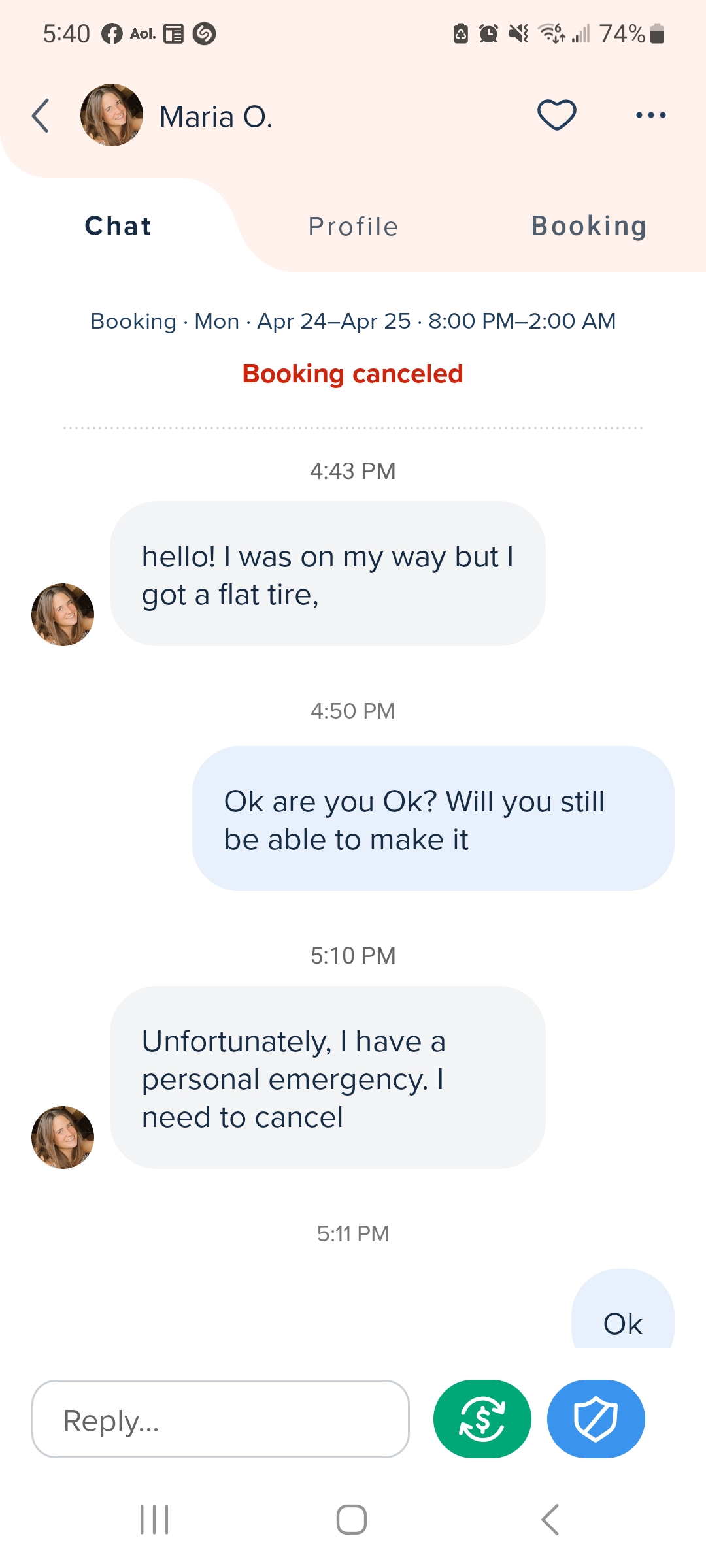This screenshot captures a detailed view of a conversation between a user and someone named Maria O. on a smartphone interface.

In the top left corner of the screen, Maria O.’s profile picture is prominently featured. She has blonde hair, is tilting her head slightly to the left, and is looking directly at the viewer with a smile. Next to her profile picture, on the right, are a heart icon followed by three horizontal dots, likely representing additional options.

The top left corner of the screen also shows the time as 5:40, while the battery level on the top right indicates 74% remaining. Below Maria O.'s profile picture, there are three tabs: "Chat" on the left, "Profile" in the middle, and "Booking" on the right. The "Chat" tab is highlighted in white, indicating it's the current active tab.

The conversation takes place within the "Chat" tab. At the top of this section, there’s a heading that reads: "Booking, Monday, April 24th to April 25th, 8 PM - 2 AM," followed by a status update that says, "Booking cancelled." 

The chat begins with Maria O.’s message: "Hello, I was on my way but I got a flat tire." The user responds with concern, asking, "Okay, are you okay, will you still be able to make it?" Maria O. replies, "Unfortunately, I have a professional emergency, I need to cancel." The user concludes the chat with, "Okay."

This detailed account encapsulates the entire essence of the conversation and the surrounding interface elements.